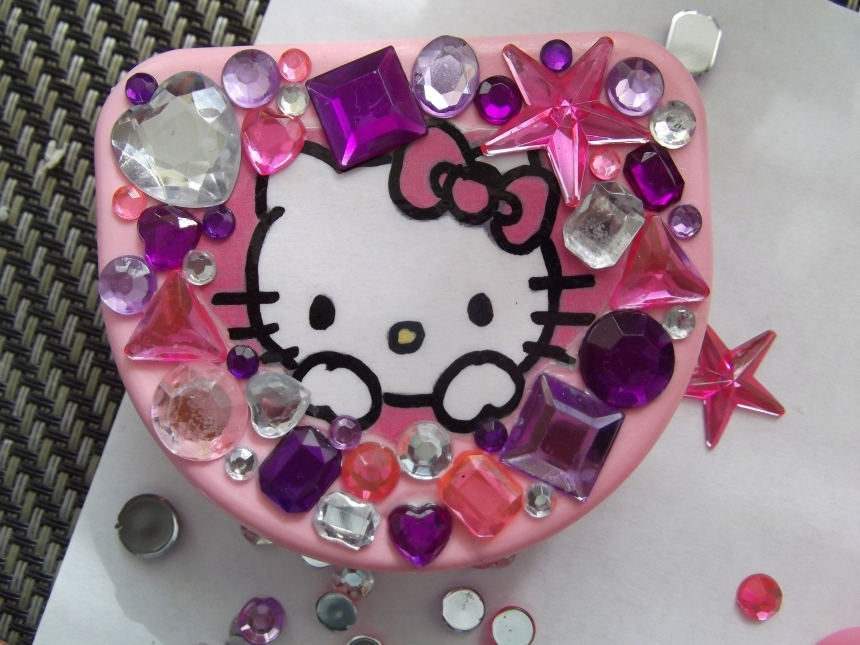This photograph showcases a vibrant piece of children’s artwork featuring a pink, shield-like container, likely representing a Hello Kitty box, set against a primarily white background with a black and cream-colored surface at the corner. The artwork is viewed from above, emphasizing its decorative nature. At the heart of this creation is an image of the iconic Hello Kitty character, distinguished by her white face, pink bow, and yellow nose. Surrounding Hello Kitty are an assortment of glued gemstones in various shapes and sizes, predominantly in hues of purple, pink, and white. These faux jewels, which include stars, squares, and ovals, enhance the whimsical feel of the piece. The placement of the stones creates a radiant, jewel-encrusted effect, making the entire artwork shimmer and draw attention.